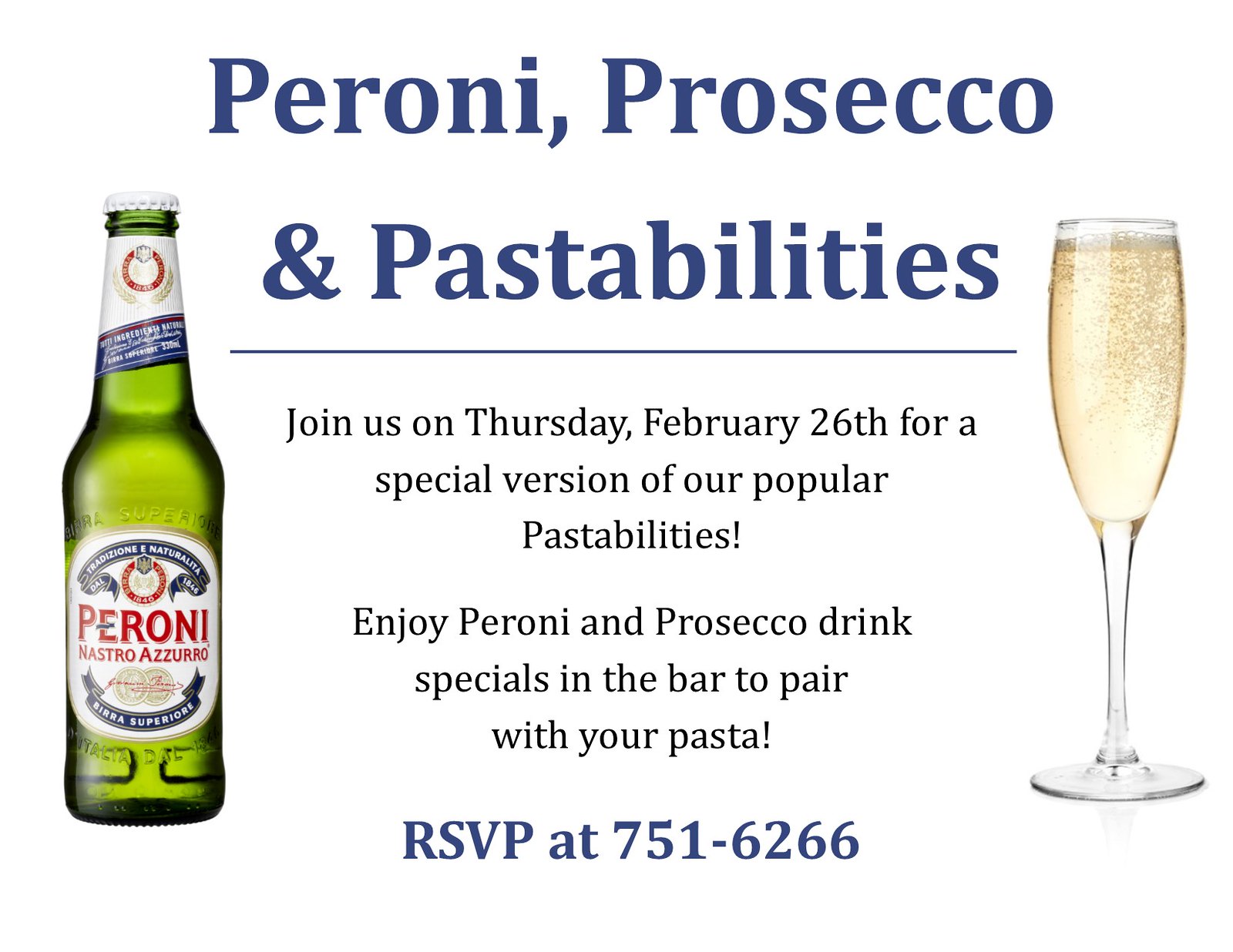This image appears to be an advertisement for a restaurant event, likely designed for social media or their website, set against a white background. Dominating the top in large blue letters is the text "Peroni, Prosecco, & Pastabilities." On the left of the image, there's a green bottle of Peroni beer, featuring a white screw cap and the label "PERONI" in large red capital letters. On the right, there's a champagne glass, filled to the top with champagne. Between these elements, in bold blue print, is the primary event title: "Peroni, Prosecco, & Pastabilities." Below a long blue line, smaller black text reads: "Join us on Thursday, February 26th for a special version of our popular Pastabilities! Enjoy Peroni and Prosecco drink specials in the bar to pair with your pasta." At the bottom, in large blue text, it instructs: "RSVP at 751-6266."